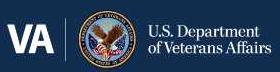The image is a horizontal rectangle with a dark navy blue background. On the left side, there are bold, white, capital letters spelling out "VA." A very thin white vertical line separates the "VA" from a round patch that features an eagle intertwined with the colors of the American flag—red, white, and blue. The patch is somewhat unclear due to the small size and blurriness of the image. The background of the patch is a light sky blue, encircled by a black ring and an outer gold border. To the right of the patch, the text "U.S. Department of Veterans Affairs" is written in white, with periods following the "U" and "S."